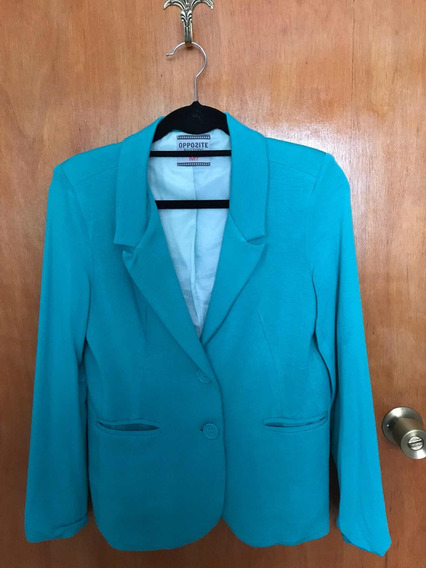In this image, a woman's turquoise blazer with double buttons and pockets is hanging on a black hanger with a metal hook. The hook is affixed to the back of a lightly stained wooden door, which features a silver cylindrical doorknob with a lock situated on the lower right side. The blazer, tagged with the brand name "Oppozite," has a darker blue exterior compared to its lighter colored lining. The collar is folded down, and the blazer appears somewhat frumpy around the sleeves. The jacket is buttoned and a tag is visible inside at the top. The door is illuminated near the right shoulder of the blazer, enhancing the texture of the wooden surface.